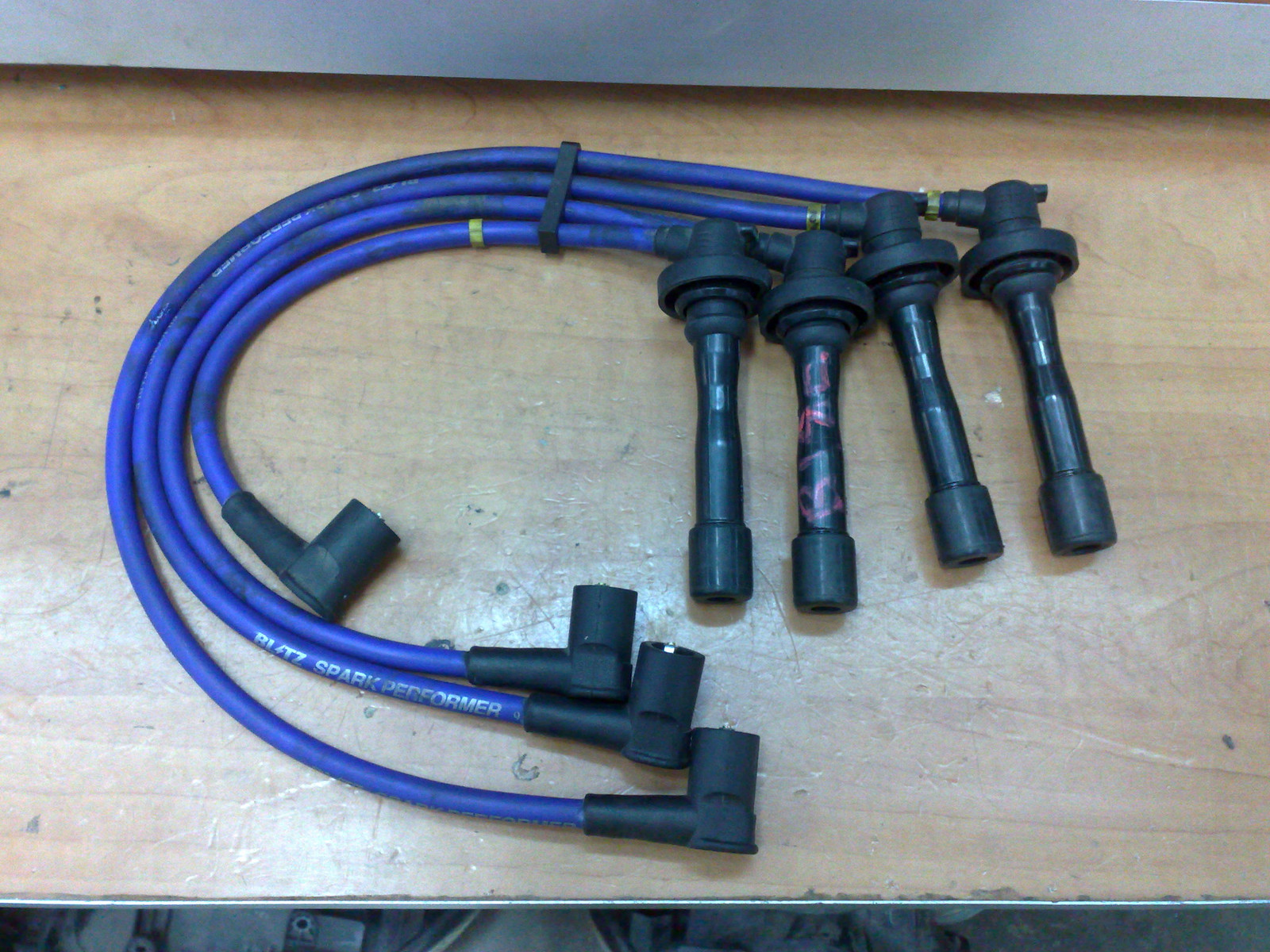In this photograph, we see a set of four blue rubber tubes, each bending into a curve, and secured together with a black clip. These tubes, which appear to be part of a device possibly related to spark plugs, feature black cylindrical ends designed for connections or air input, each topped with a cap. One end has a long, sleek black cap, while the other side has a shorter black component with an L-shaped extension branching off. The blue tubes are laid out on a light brown wooden table, visibly worn with dark scratches, stains, and various black marks. In the background, a white wall is partially visible, and the bottom of the image shows what appears to be a stone floor, suggesting a garage or workshop setting. The tubes seem to be products from a brand named Blitz Spark Performer, which is indicated by some text in the photograph. This detailed setup likely aims to display the device, possibly for sale on platforms like Amazon or eBay.